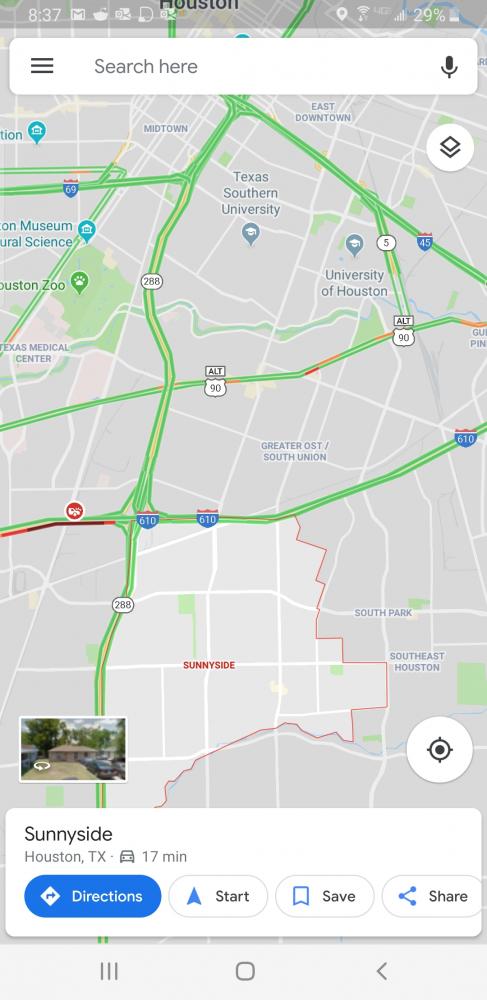The image is a screenshot from a smartphone displaying a Google Maps interface. At the bottom, it prominently features the locale "Sunnyside, Houston, Texas," along with an icon of a car and an estimated travel time of 17 minutes. Below this, there are several interactive buttons: a blue button labeled "Directions," a "Start" button, a "Save" button, and a "Share" button. 

The underlying map highlights the Sunnyside area in red and shows its surroundings, including landmarks such as Texas Southern University, the University of Houston, East Downtown, Midtown, Hudson, Houston Zoo, Greater OST, and South Union. Major highways like Interstate 45 and Interstate 610 are also visible. 

In the lower left corner of the map, there is a small thumbnail image of a house, which likely indicates either the starting point or the destination of the map's user. 

At the very bottom of the screenshot, the typical navigation buttons of an Android phone are visible: the 'back' button, the circular 'home' button, and the 'overview' button (represented by three horizontal lines). 

Overall, the screenshot captures a comprehensive map display on a smartphone, enriched with various navigational and location-specific details.